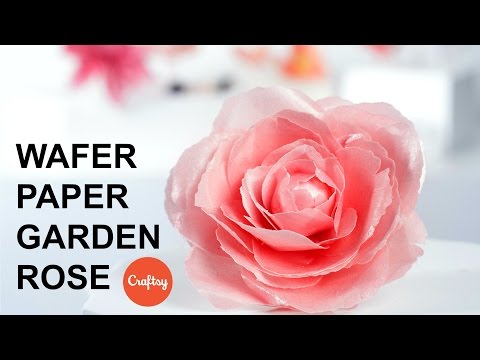The image is a rectangular, letterbox-style ad with black bars on the top and bottom, creating a cinematic effect. The main focus is a large, intricately crafted pink rose made from wafer paper, which prominently occupies most of the white background. This rose is beautifully detailed, with its outer petals in soft pink that gradually transition to a deeper red along the edges and then back to a soft pink in the very center. To the left of the rose, the phrase "wafer paper garden rose" is displayed in black capital letters, stacked in four lines. On the right side of the image, there's a red circle with the word "Craftsy" written in white cursive font, indicating the brand or source of the rose. The background is slightly blurred, with hints of other colorful elements and shapes, including a dark pink flower and possibly some black dots and an orange flower, adding depth and context to the scene.